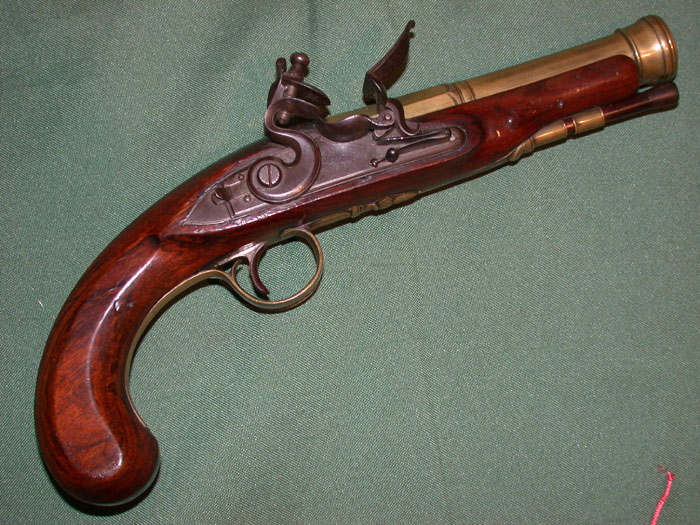This image is a detailed photograph of an antique flintlock pistol, positioned against a gray-green fabric background. The pistol features a well-worn, reddish-brown wooden handle that resembles mahogany, adding a sense of deep, rich color to the piece. The trigger and striker mechanism are made from ornate brass and darker metal elements, showing intricate craftsmanship. The main barrel of the pistol, which is somewhat large and slightly flared at the opening, is composed of brass that gives off a copper-gold hue. The entire gun, including its brass and metal components, exudes a sense of age and historical significance, likely dating back to the 17th or 18th century. Despite its antiquity, the pistol appears to be in remarkably good condition, suggesting careful preservation over the years. The hefty and robust design, with its combination of metals and wood, underscores the functional elegance of historical weaponry.